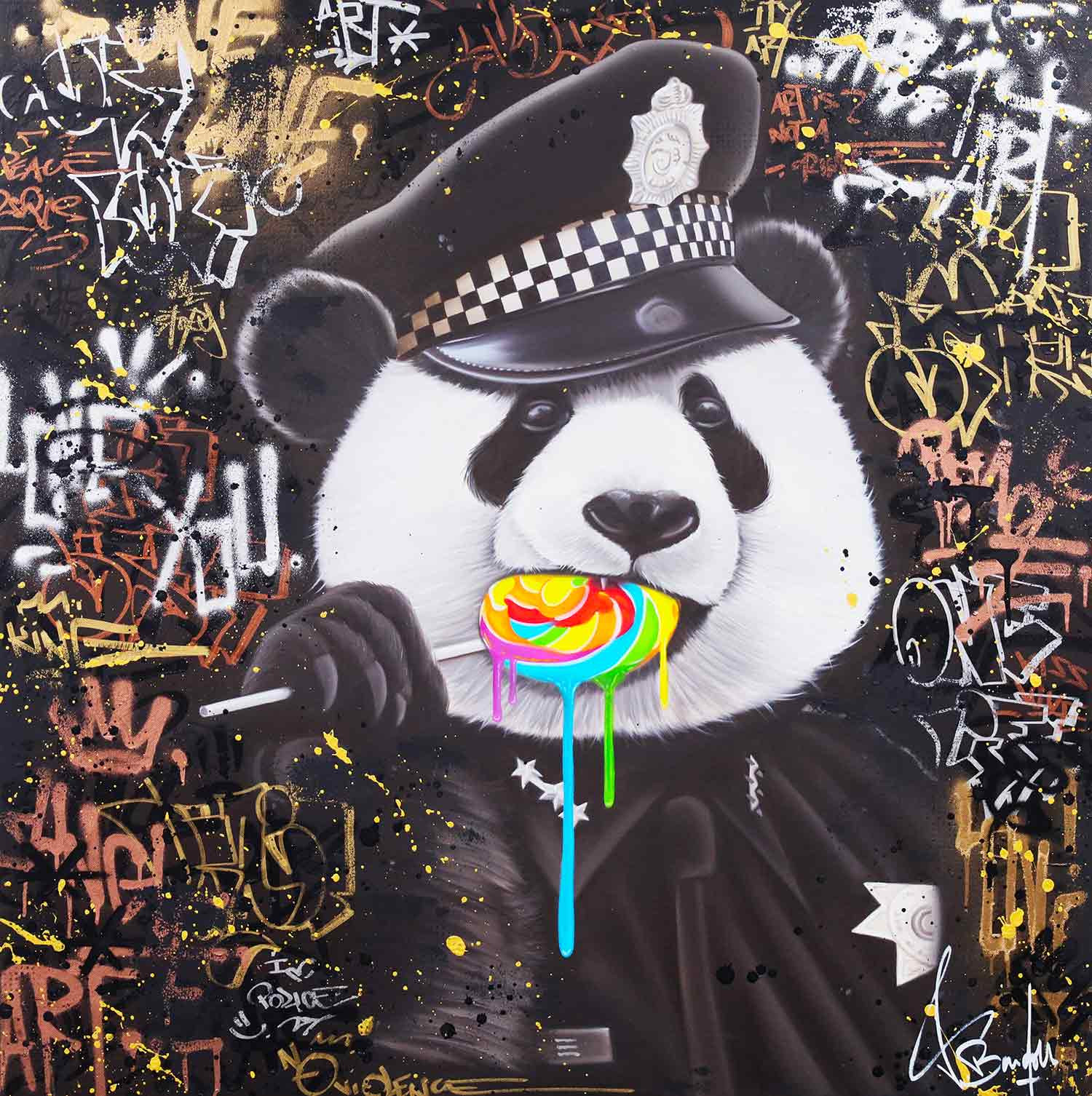This abstract painting, potentially computerized or on a physical wall, features a striking portrayal of a panda bear dressed as a policeman. The panda, depicted in black and white, dons a detailed police uniform, complete with a black cap adorned with black and white checkers and a police badge. The panda is savoring a large, rainbow-colored lollipop with one paw, from which melting candy drips in vibrant colors of purple, blue, green, and yellow. Surrounding the panda is an array of graffiti-like text, mostly illegible and perhaps not in English. The artist's name, which appears to be something akin to "BAUN," is marked in white in the lower right corner. This eclectic piece blends traditional painting with elements of street art, making it a captivating visual experience.